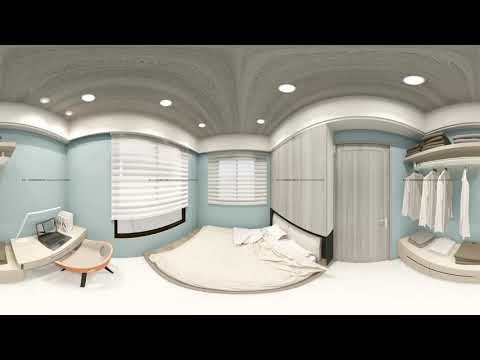The image depicts a panoramic photograph of an indoor space, possibly a bedroom or studio apartment, characterized by walls painted in a light seafoam greenish blue. The use of a curved lens makes the walls appear rounded, adding a unique visual aesthetic. The ceiling is gray with integrated lighting. Thick black rectangles crop the top and bottom of the wide, rectangular image.

Key elements in the room include several windows with large sheer white blinds. In the center, a white bed lies low on the floor, covered with additional blankets and accompanied by two white pillows at its headboard. Above the bed is a set of gray wooden cabinets. 

To the right of the image, a clothing rack displays four identical white shirts hanging in a row. Adjacent to this is a tall gray wooden door. The left side features a peach-colored chair with black legs, and a gray laptop with its lid open sits in front of the chair. The room is devoid of any people, words, or numbers. Overall, the room exemplifies a modern, minimalist aesthetic through its clean lines, color palette, and functional furnishings.